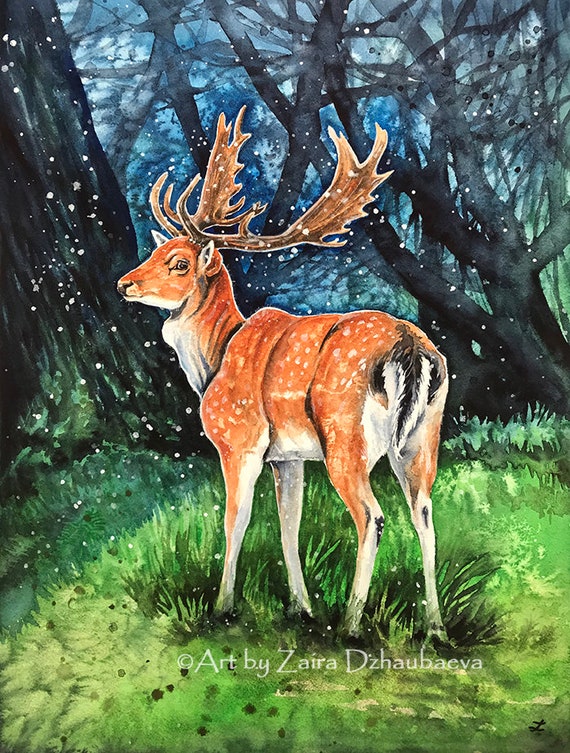This is a beautifully detailed watercolor painting by Zaira Dzhaubaeva, featuring a majestic buck standing in a grassy meadow surrounded by a dark, dense forest. The deer, with its large and intricate antlers, is captured in a moment of alertness, gazing back over its left shoulder at the viewer. Its fur is a warm brownish-orange adorned with white spots, while its underbody, front legs, and the back of its legs are highlighted with white. The tail, a striking black with white edges, adds to the animal's distinct features. The scene is set under a softly lit sky, painted in shades of blue, suggestive of either dawn or dusk, and is imbued with a sense of serenity as snow gently falls, adding a whimsical touch. The grass beneath the deer ranges from light to dark green, hinting at the nuanced brushwork. Trees, painted in dark hues of black and brown, with bare branches, frame the background, enhancing the focal point of the painting. Near the bottom right corner, the artwork is signed "Copyright Art by Zaira Dzhaubaeva" in white text.